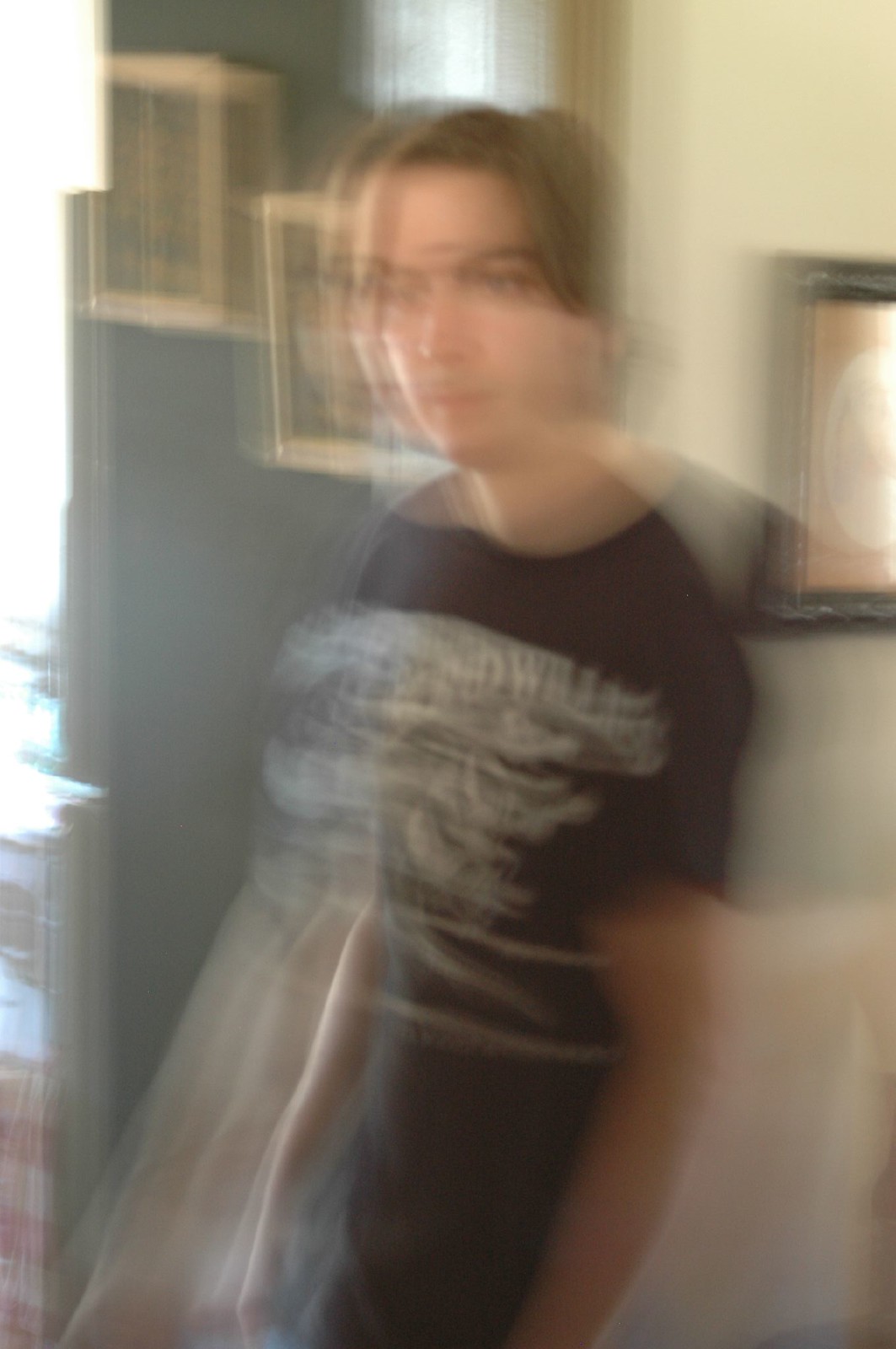This photo, suffering from extreme motion blur akin to double or triple exposure, depicts a young man standing inside a home. His short brown hair, possibly styled in a mullet, reaches down to his chin. He is wearing a black short-sleeve t-shirt adorned with a vague white design, possibly containing comical elements. The scene is set against two different walls. To his left, the wall is off-white with a black-framed picture or painting. In contrast, behind him and to his right, the wall appears dark gray or dark green, featuring two picture frames with white borders. The man, appearing to be in his early 20s and of European descent, is captured in a doorway amidst an array of framed photographs, though the extreme blur obscures the finer details.